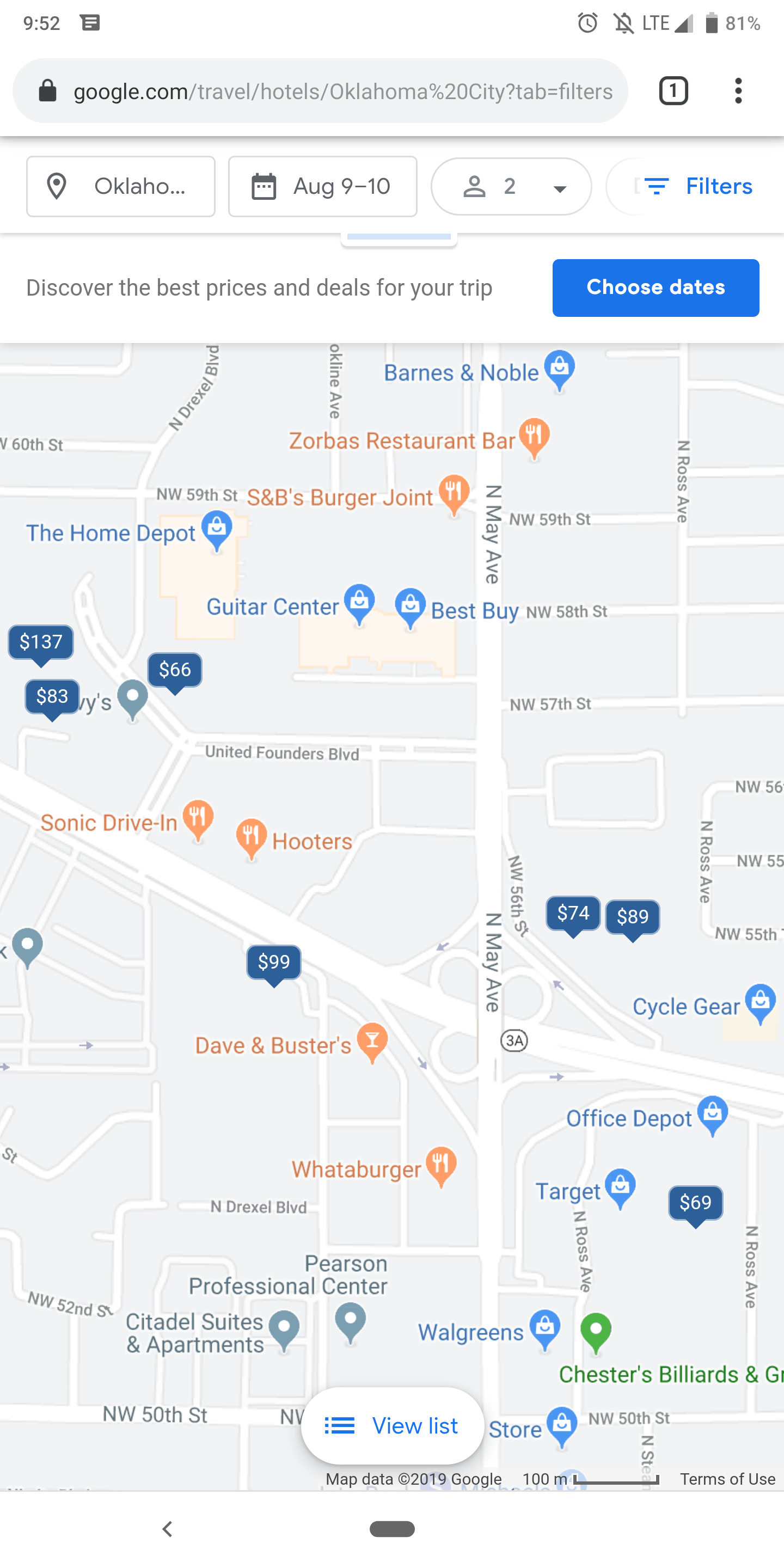The image depicts the screen of a smartphone displaying a Google search page for hotel deals in Oklahoma City. The top status bar shows the time as 9:52 with a signal indicator showing three to four bars, an LTE indicator, a muted notification bell icon, and a battery level of 81%.

At the top of the display, a gray search bar includes a black padlock icon followed by the URL: "google.com/travel/hotel/Oklahoma%20City?tab=filters." Below the search bar, the screen indicates the search parameters: "Oklahoma, August 9th through 10th, two people" with corresponding icons for location, calendar, and people. To the right of these details, a blue "filters" label is visible.

A banner on the left reads, "Discover the best prices and deals for your trip," above a blue button labeled "Choose dates." Below this, a large light gray map is populated with orange markers indicating restaurants and blue markers for stores. Some of the listed restaurants include Zorba's Restaurant Bar, S&B's Burger Joint, Sonic Drive-In, Hooters, Dave & Buster's, and Whataburger. Stores displayed include Barnes & Noble, Guitar Center, Best Buy, The Home Depot, Target, and Walgreens. Numerous other locations, such as Citadel Suites and Apartments and Pearson Professional Center, are also marked on the map. Roads and streets are clearly labeled, providing a comprehensive view of the area. 

At the bottom, a partially obscured banner offers a "View list" option, depicted with three horizontal blue lines.